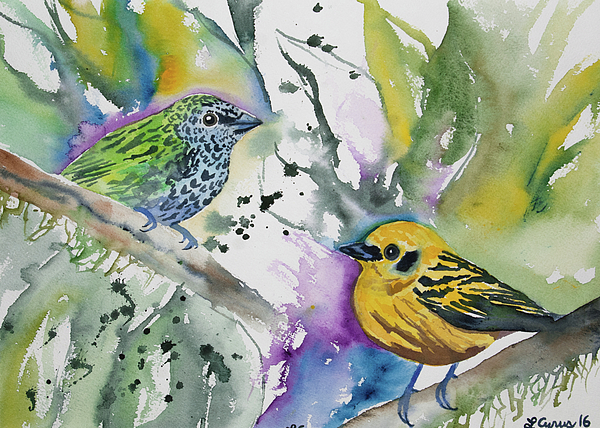This rectangular watercolor painting presents a vivid scene with two birds perched on different branches of the same tree. The background is a blend of abstract and chaotic splashes of color, predominantly greens and yellows, set against a white backdrop that peeks through in places. 

The bird in the lower right corner is primarily yellow with black accents on its wings and a black beak. It stands on a branch angled from the bottom to the right side of the painting. Its circular black eye and left side profile are prominently visible as it faces upwards and to the left. The artist has signed the piece in the lower right corner with an elegant cursive that reads something like "El Caruso 16" or "LG something" followed by "16," indicating it was created in 2016.

The second bird, which occupies the upper left corner, is characterized by its blue face and chest with black feather markings, and green wings accented with darker green and grayish patterns. This bird stands on a branch that angles from the lower center to the upper left of the image. Like the first bird, it gazes in the direction of its companion, suggesting a sense of communication between the two.

The tree branches they rest on intersect at points, weaving through the vivid splashes of color that possibly represent leaves or flowers. Despite the abstract nature of the background, the painting's emphasis on the detailed plumage and the expressive posture of the birds creates a captivating focal point.